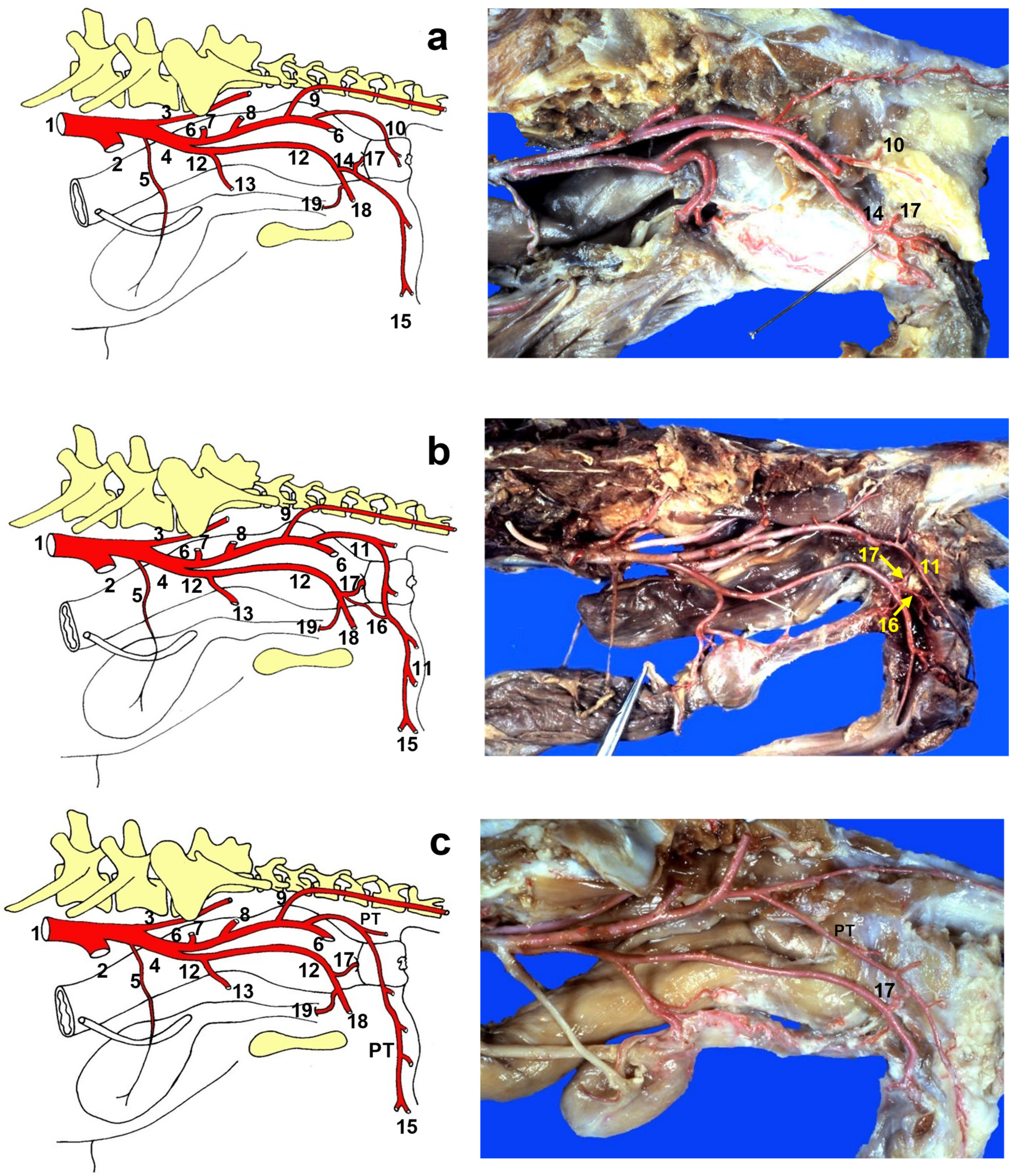The image depicts a detailed analysis of an unborn animal, likely a fetus, accompanied by anatomical diagrams. On the left side, there are three labeled diagrams, A, B, and C, which display the spinal column, blood vessels, and various other parts of the body in distinct colors: yellow for bones, red for veins, and other shades for different tissues. These diagrams are meticulously numbered to correspond to specific body parts. On the right side, three corresponding images of the actual fetus are shown against a bright blue background. These real-life photos reflect the anatomical details illustrated in the diagrams, featuring a gray, yellow, and red creature that appears to have died in utero. The images show the dissected fetus in different positions, possibly part of an autopsy to understand why the animal was not viable.